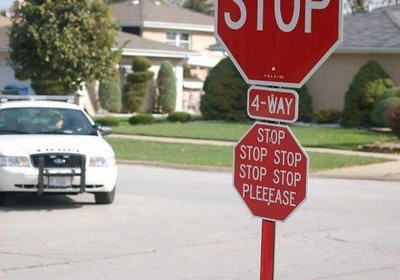The image captures a bright, sunny day in an affluent residential neighborhood marked by meticulously manicured lawns, neatly trimmed bushes, and gracefully landscaped trees. Front and center, slightly to the right, stands a traditional red octagonal stop sign with the word "STOP" and a white stripe around its edge. Beneath it, a smaller sign reads "FOUR-WAY" in white letters on a red background, and directly below this is another, smaller stop sign which reads "STOP, STOP, STOP, STOP, PLEASE" in white letters on a red background, similar to the top sign. The intersection, partially out of view, is being approached by a white police car with a push bumper making a right turn. The officer inside, of European descent, is visible through the window. In the background, several expensive two-story homes are visible, showcasing lush green lawns, carefully maintained shrubs, and a backdrop of deciduous trees. This well-tended and serene setting gives the impression of a safe and orderly neighborhood.